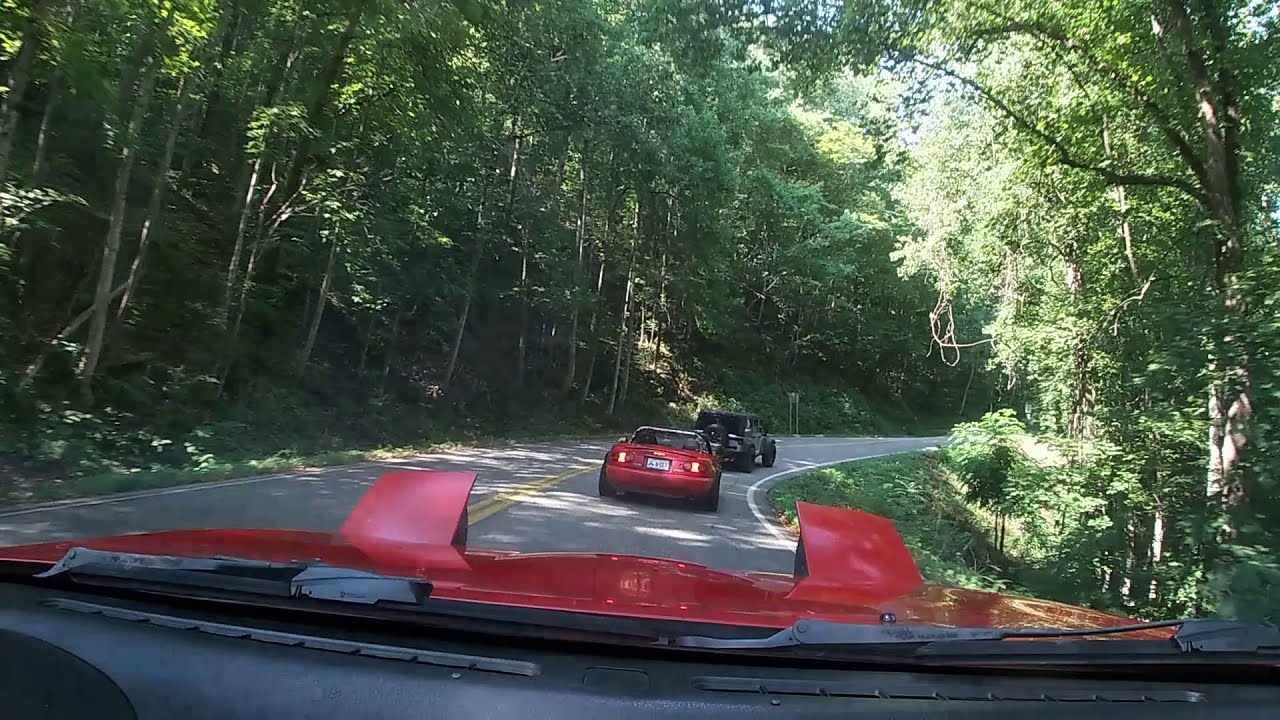In the photograph taken on a bright sunny day, the view is from the interior of a red sports car with raised headlight covers, suggesting it's an older model. The dash and a bit of the hood are visible, revealing the partially lifted headlights. The car in front is a red convertible, likely a Corvette, with its rear taillights on, suggesting it might be braking. Leading this small convoy is a gray or black Jeep, which has a distinctive, boxy shape. They are navigating a winding, two-lane road that meanders through a densely forested area. Trees rise steeply on the left side, forming a hilly embankment, while the right side of the road slopes downward, similarly covered with lush trees. The trees obscure much of the sky, except for a small visible section in the center top to the top right corner, emphasizing the seclusion of the wooded area. The road curves gently to the right before disappearing from view. The shadows cast by the trees suggest it is mid to late in the day, adding to the serene atmosphere of the forested journey.